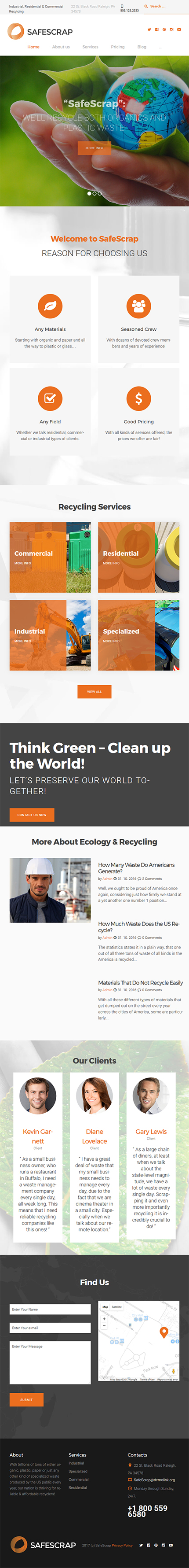The image depicts a screenshot of a website that is challenging to read due to an improper aspect ratio, causing all text and images to appear stretched and distorted. The website seems to focus on environmental and recycling topics, as suggested by the central gray banner bearing the text "Think Green, Clean Up the World." The background of the page is predominantly white and light, creating a clean aesthetic. At the very top, there is a banner image featuring a hand holding the Earth, symbolizing care for the planet. Below this are testimonials from three different individuals, each accompanied by their photographs and a brief description of their comments, though these are unreadable due to the distortion. Further down, the webpage provides input fields for user interaction or comments.